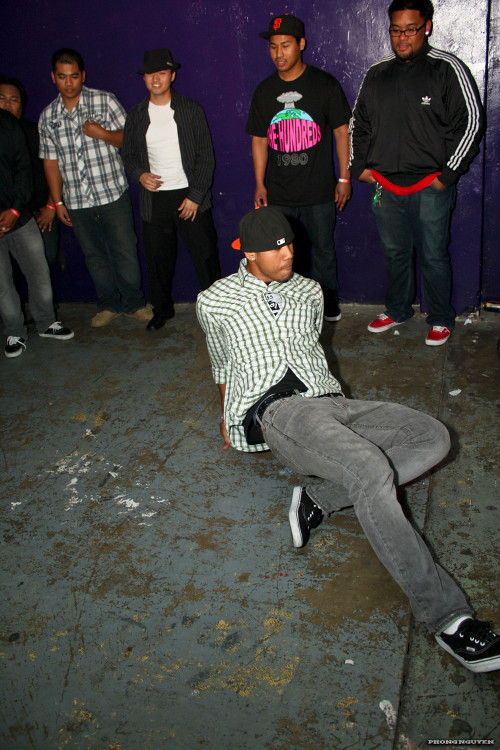In a vertically oriented photograph, a breakdancer of apparent Mexican descent is captured mid-performance on the floor. He is engaged in a dynamic spinning move, with his hands positioned behind his back. The dancer is adorned in a white checkered shirt, black pants, and black Vans sneakers, complemented by a backward-facing baseball cap. Lively onlookers, totaling five, stand against a vivid purple wall, each sporting different expressions as they watch the performance unfold. Among the spectators, one individual wears glasses, another sports a black overcoat with sleeve stripes, and another dons a t-shirt with a "100" graphic. The remaining onlookers are dressed in casual attire, including a light black jacket over a white t-shirt, a black and white checkered shirt, dark pants, blue jeans, and various sneakers. The scene, likely set in a building or club, presents a captivating exhibition of hip-hop dance.